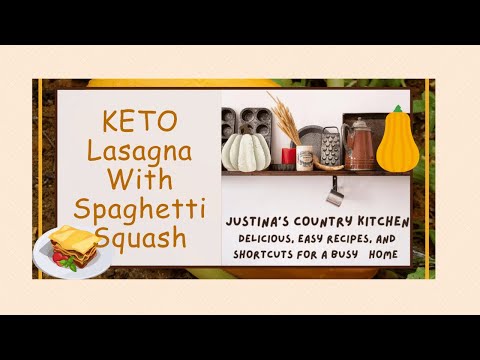This kitchen-themed artwork, designed for display, showcases the phrase "Keto Lasagna with Spaghetti Squash" in a muted mustard yellow font against a creamy white background. Dominating the upper portion, this inviting message is complemented by an illustration of a lasagna dish in the bottom left corner. Adjacent on the right, a shelf displays an assortment of culinary items including muffin tins, a rustic pumpkin planter, another decorative pumpkin container, a sprig of wheat, a pan, a seasoning holder, a cheese grater, and what appears to be a vintage coffee urn. Below these visual elements, the caption "Justina's Country Kitchen: Delicious, Easy Recipes and Shortcuts for a Busy Home" is neatly written, encapsulating the warm, homemaker vibe. The artwork is framed by a light tan and wooden border adorned with greenery, leaves, and branches, enhancing its cozy, country-style appeal.